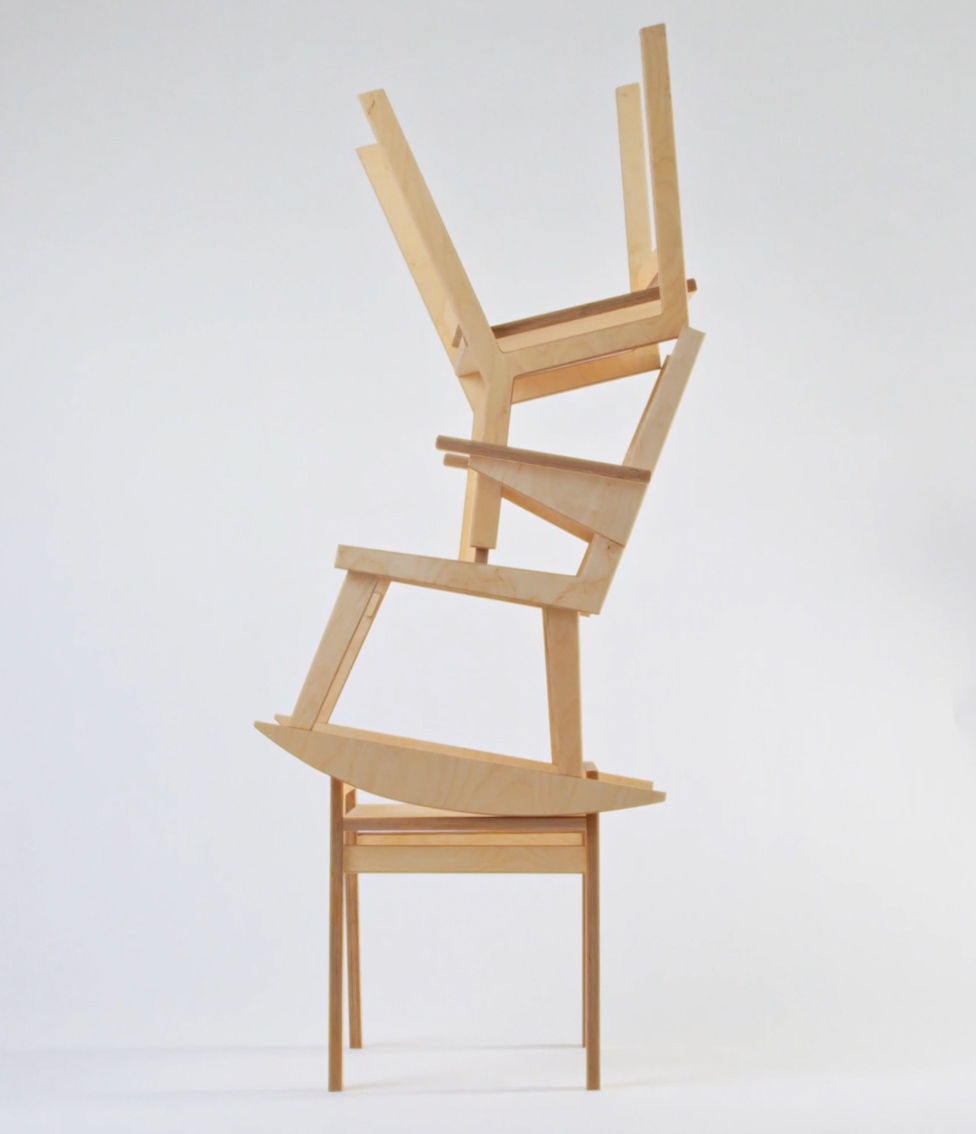The photograph captures three wooden chairs stacked in a visually intriguing arrangement against a pristine, all-white backdrop, likely within a photography studio. The composition features a light brown, almost yellowish, wooden chair standing upright on the floor. Balanced atop this is a wooden rocking chair, and crowning the stack is a normal wooden chair, flipped upside down, with its four legs pointing skyward. The chairs appear to be laser-cut and meticulously arranged in an atypical, linear fashion, drawing the viewer's attention to their precarious yet harmonious balance.